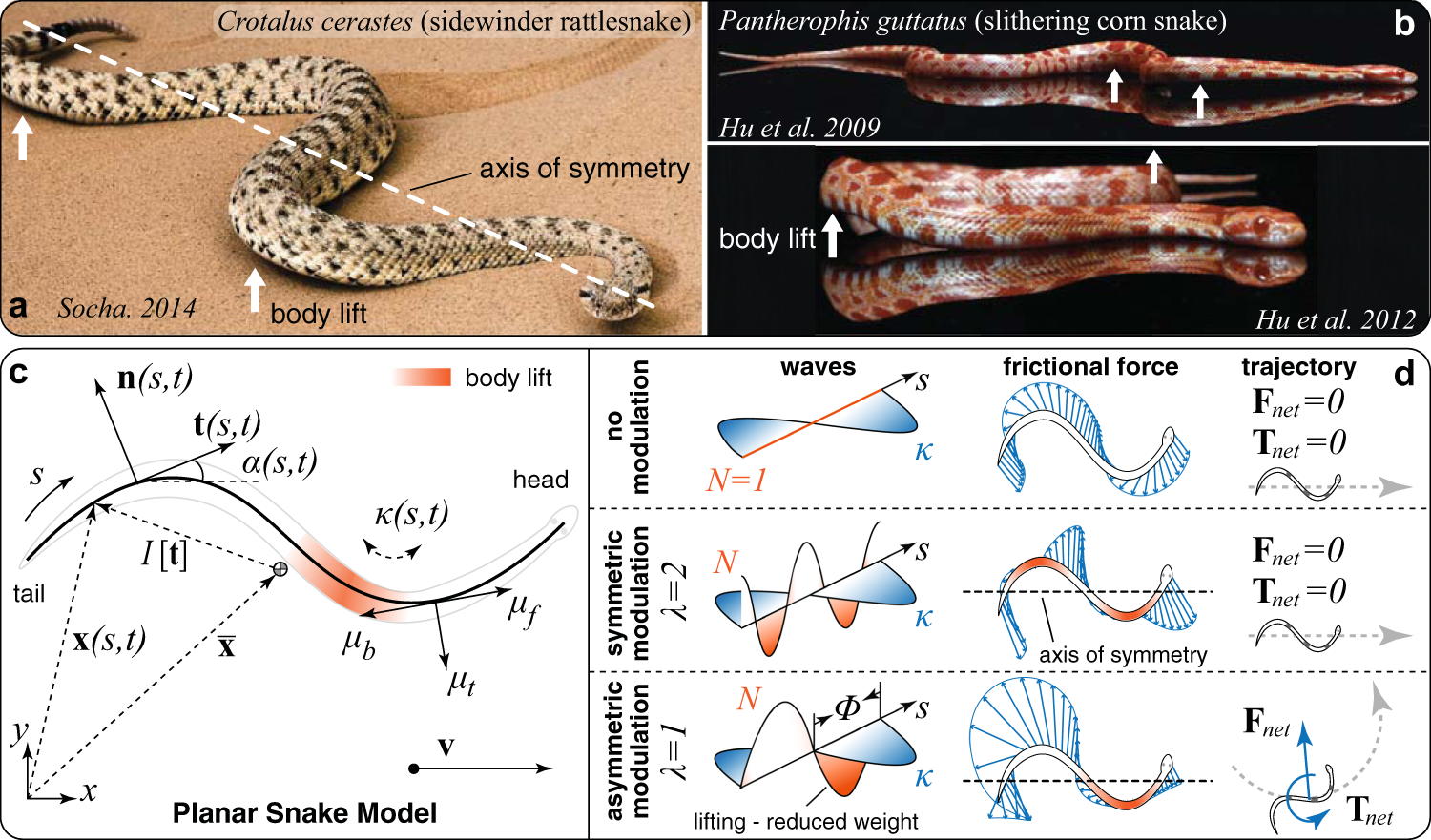This detailed image from a textbook is divided into an upper and a bottom portion, each providing rich informational content about snakes. The upper portion is further split, with the top left showcasing a photograph of a sidewinder rattlesnake (Cotalis ceratus) by Socha (2014). A dotted diagonal line, labeled as the axis of symmetry, runs from the snake's tail to its head, illustrating the snake's movement pattern.

Adjacent to this, on the top right, are two images of a Pantheropus guttatus (Slytherin corn snake), taken by Hugh et al. (2017). These images display the snake's body lift with arrows marking each section of the snake's body. The top image shows the snake from a side view while the bottom image focuses on the details of its undulating movement.

The bottom portion of the image is labeled "Planar Snake Model" and features geometric illustrations, including lines, waves, and triangles. It details different mathematical formulas and concepts related to the snake's movement, specifying areas such as frictional force and trajectory. This section is further divided into three rows, each explaining various aspects of the snake's locomotion through diagrams and text.

Overall, the top portion uses color photography to visualize the snakes and their movements, while the bottom portion employs illustrative diagrams to break down the mathematical models of these movements.